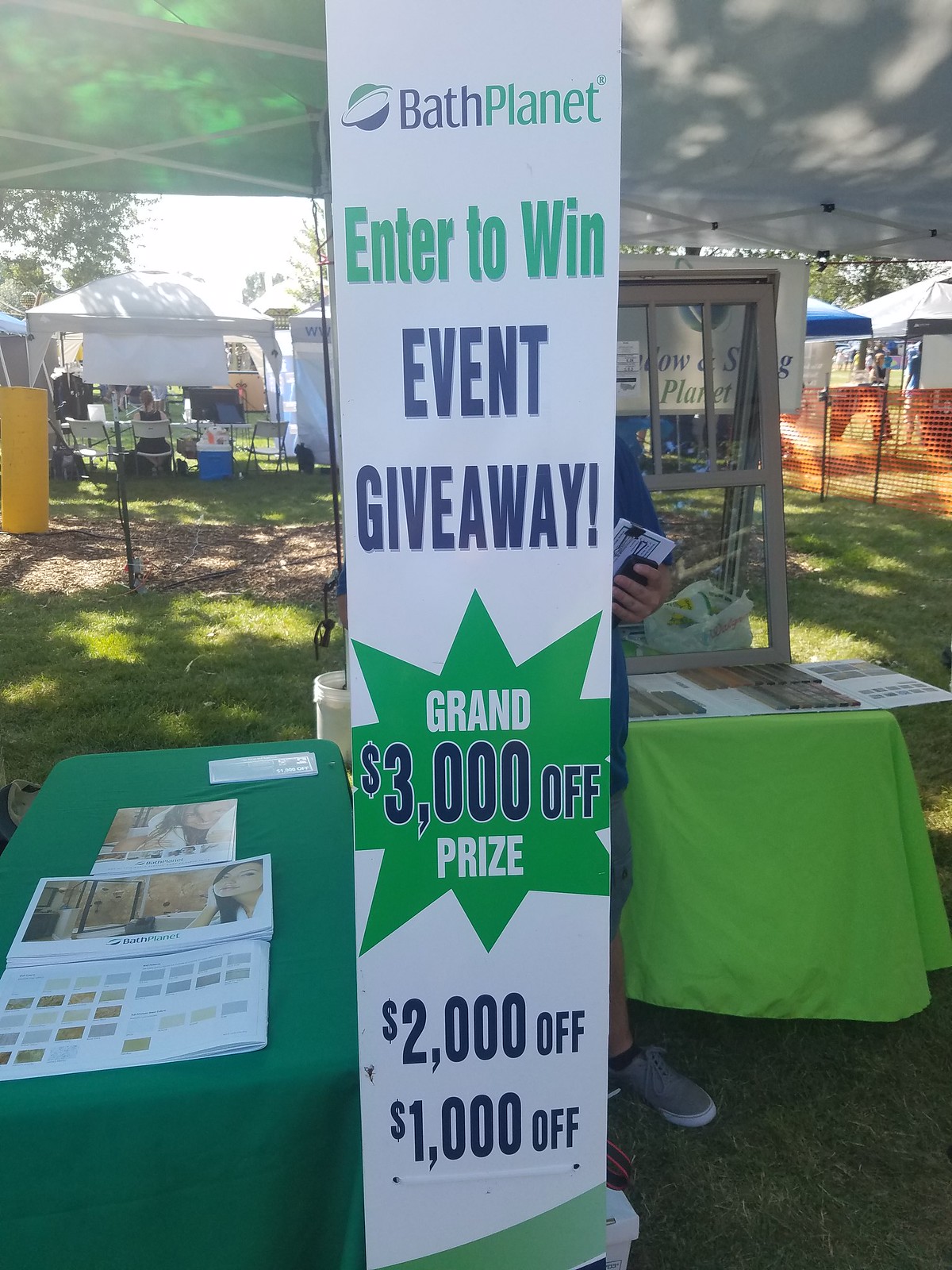The image captures a bustling outdoor event, likely a farm fair or carnival, featuring a prominent vertical banner advertising a giveaway by Bath Planet. The sign is centrally placed in the foreground, with the top of the banner displaying "Bath Planet" in a navy and green color scheme. Below, the text reads "Enter to Win" in green, and "Event Giveaway" in navy. A vibrant green starburst highlights the grand prize of "$3,000 Off" in navy letters, flanked by the words "Grand" and "Prize" in white. Beneath it, additional prizes of "$2,000 Off" and "$1,000 Off" are listed in navy font.

To the left of the sign stands a table draped in a dark green cloth, showcasing three different types of pamphlets. On the right, another table covered in light green holds wood or tile samples and is backed by a sample window. A man, identifiable by his hand, shoulder, and a portion of his left foot, stands partially hidden behind the sign. He appears to be wearing a blue shirt and gray and white shoes.

The backdrop reveals a typical fairground scene with multiple pop-up tents, grassy areas, and scattered patches of dirt, all under a clear sky with visible trees. The tent roof covering the Bath Planet booth is faintly visible at the top of the image, providing shade to the display area.